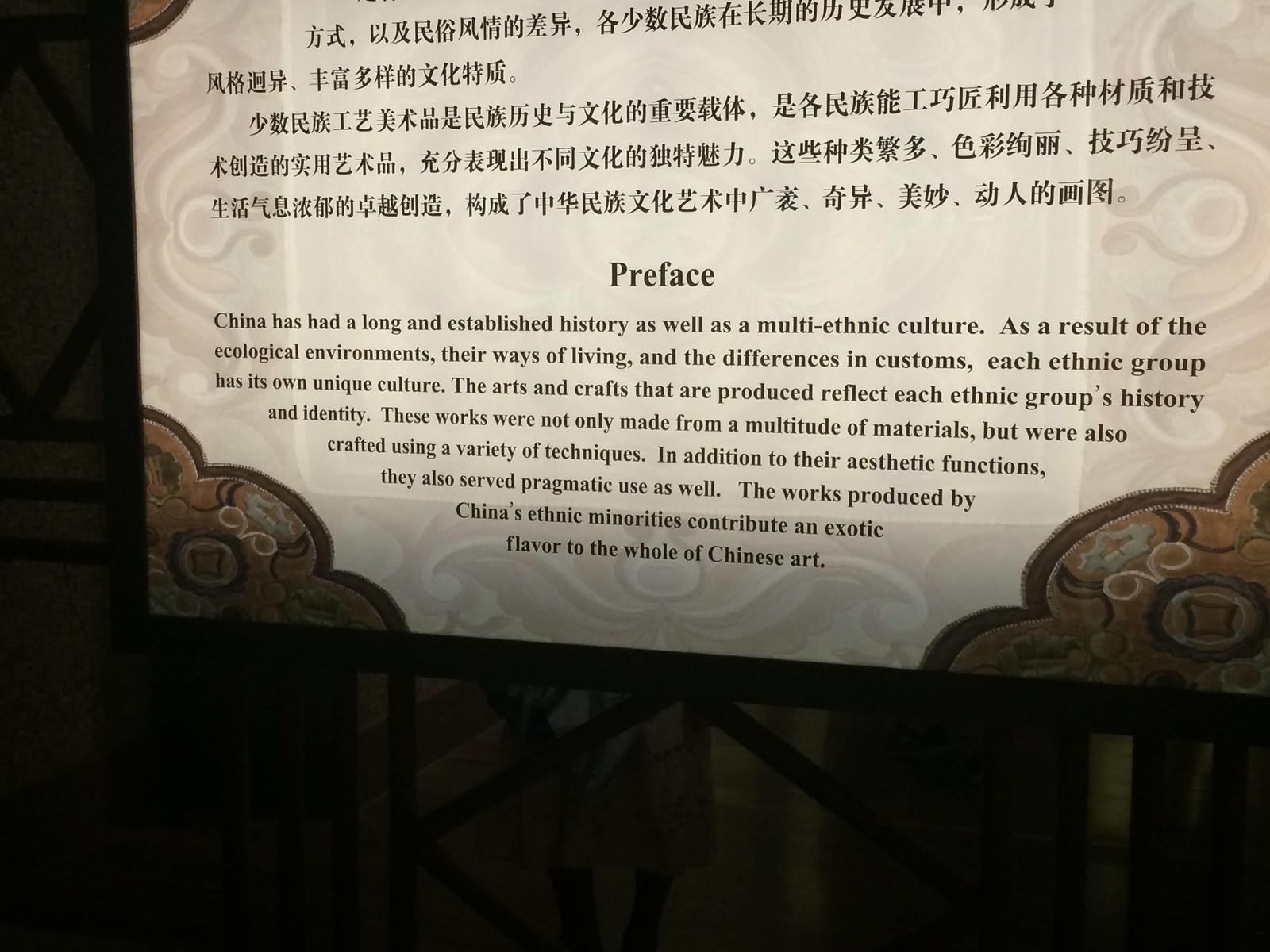The photograph depicts a dimly lit sign, resembling a certificate or display, situated in a predominantly shadowy setting with a faintly visible greyish background. The sign features an intricately designed border, adorned with a mosaic pattern that transitions from dark brown to light brown and cream, creating an elegant and somewhat antiquated aesthetic. The top section of the sign is inscribed with text in Chinese characters, while the bottom section presents an English passage starting with the word "Preface." The English text reads: "China has had a long and established history as a multi-ethnic culture. As a result of the ecological environments, their ways of living, and the differences in customs, each ethnic group has its unique culture. The arts and crafts that are produced reflect each ethnic group's history and identity. These works were not only made from a multitude of materials but were also crafted using a variety of techniques. In addition to their aesthetic functions, they also served pragmatic uses as well. The works produced by China's ethnic minorities contribute an exotic flavor to the whole of Chinese art." This sign appears to be an informative display on Chinese art and its multifaceted cultural heritage.